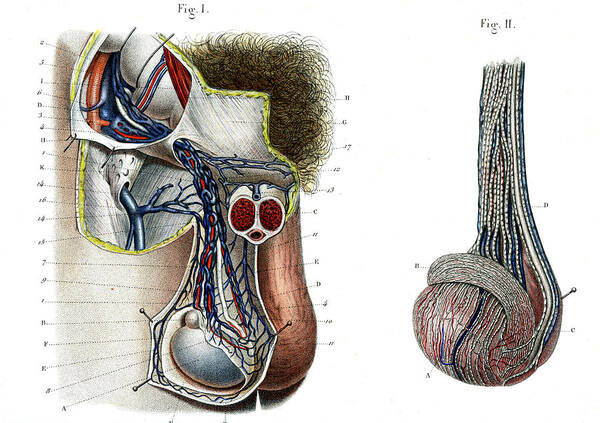The image is a detailed medical illustration against a solid white background, featuring two side-by-side figures labeled "Figure 1" and "Figure 2." Figure 1 appears to depict the internal anatomy of a human body, with various organs and a complex network of veins, both red and blue. There are numerous labeled parts, annotated with single letters such as G, H, B, C, and F, connected by lines to different sections of the drawing. The illustration seems to have cutaway views, showing detailed, fibrous structures of the organs. In Figure 2, a more external view of one of the components from Figure 1 is displayed, emphasizing the intricate and fibrous nature of the organ shown. Overall, the drawing appears meticulously detailed and anatomically informative, though the exact organs depicted are not immediately identifiable.